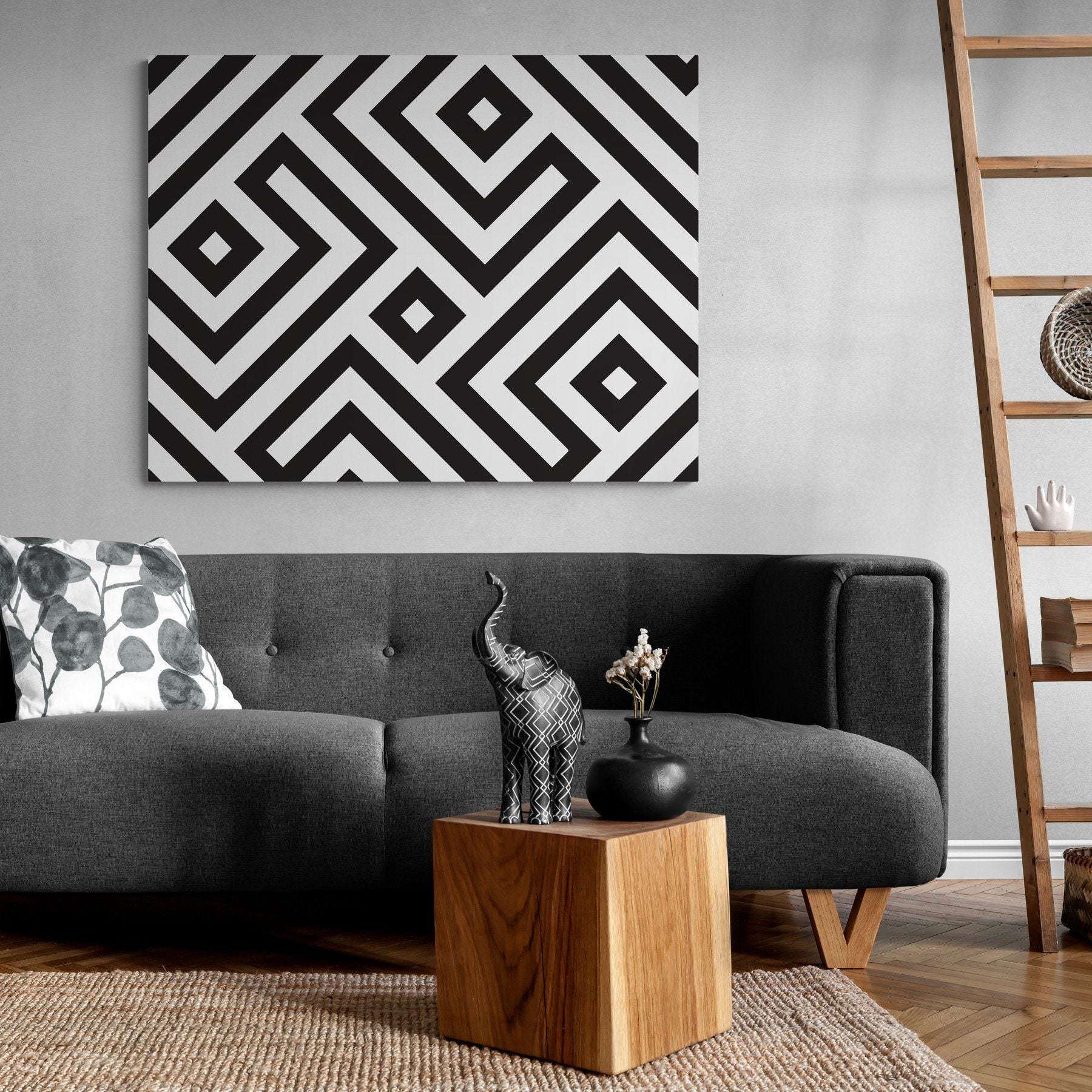This photograph depicts a stylish living room featuring a contemporary design with notable details. Central to the room is a long, dark gray sofa adorned with a white and gray pillow that has a leaf pattern. The sofa sits against a light gray wall accented with white baseboards, and prominently displayed above is a large black and white print resembling a maze or intricate geometric design.

The floor is covered with small, angled wood-grained slats, partly overlaid by a light brown, Berber-style rug. On the rug rests a wooden block coffee table showcasing distinct wood grain texture. Atop the table are two striking items: a black vase filled with flowers and a black elephant statue decorated with white diagonal patterns and an upraised trunk.

To the right of the setup, a thin wooden ladder acts as an artistic shelf, holding a ceramic hand, some books, and a pot, adding a unique touch to the room’s decor. Overall, the room's elements combine to create a cohesive, inviting space with a mix of modern and eclectic details.